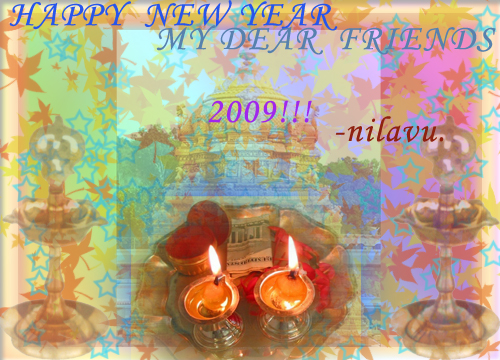This is a vibrant greeting card celebrating the New Year, adorned with an autumnal palette featuring shades of orange, green, yellow, pink, brown, and purple. At the top, in bold blue text, it says, "Happy New Year, my dear friends." Below this greeting, in purple text with three exclamation points, is the year "2009." Accompanying these celebratory messages is the word "NILAVU" in red. The card's background has a soft depiction of a dome-shaped building, possibly a Hindu temple, with intricate and faded Hindu iconography. At the foreground, two lit candles on a gold dish are prominent, flanked by unlit candlesticks. Additionally, what appears to be a five-dollar bill is placed beside the candles, all atop a metallic tray. This colorful and textured composition uniquely blends festive, cultural, and monetary symbols, capturing a moment of celebratory ritual.